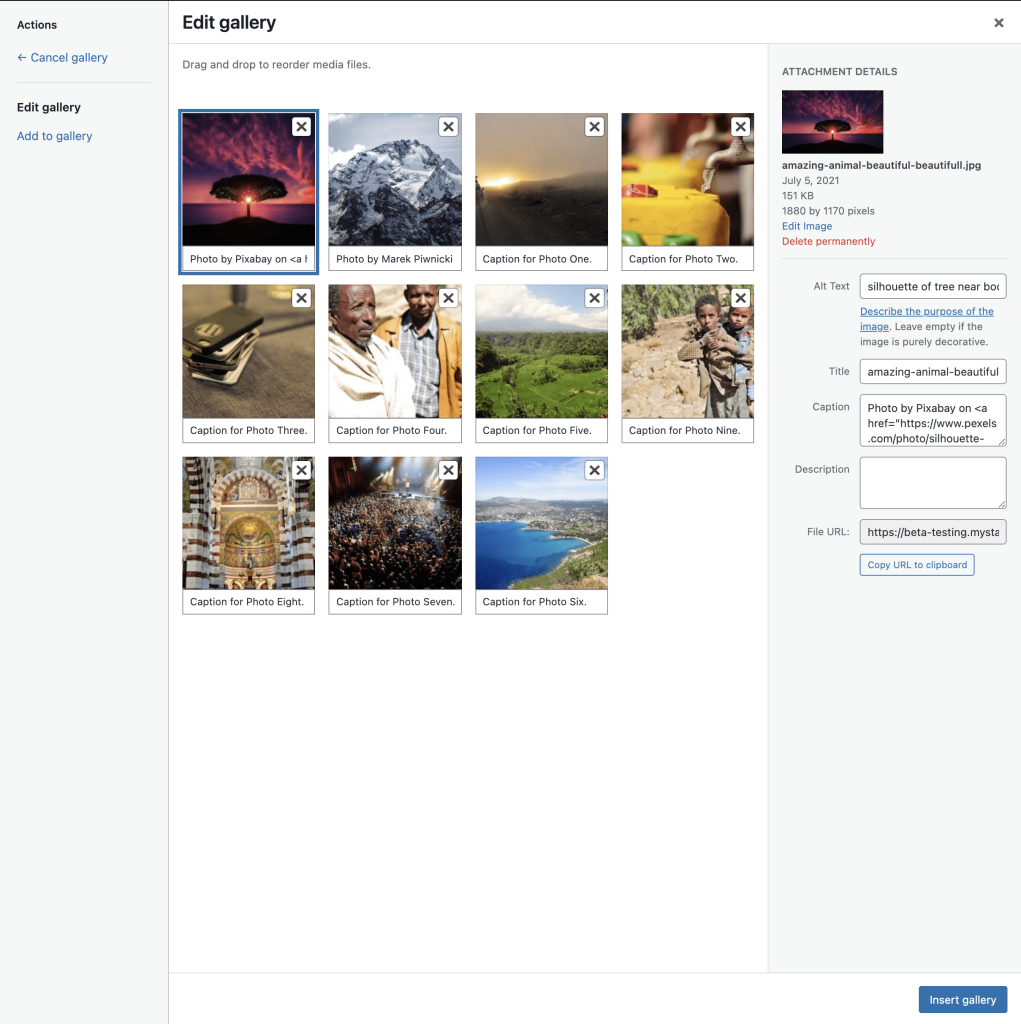On the editing gallery page, users can reorder their media files through a drag-and-drop interface. On the left-hand side, there is a menu with a series of actions: a 'Cancel Gallery' button in blue text, followed by a 'Edit Gallery' button in black, and an 'Add to Gallery' button in blue text. 

To the far right, there is a section for 'Attachment Details' for each selected photo. The details for the currently selected image, a photograph by "Pixabay," are shown here. The image depicts various natural landscapes including mountains, a stack of phones, vast grasslands, forests, and a seaside ocean. The selected photo's details are as follows:

- Title: "Amazing Animal"
- Description: "Beautiful, beautiful JPEG"
- File Size: 151 kilobytes
- Dimensions: 1880 x 1170 pixels
- Predominant Colors: Green and Blue

Below these details, there are several interactive options: an 'Edit Image' button and a 'Delete Permanently' button in red. Users also have the ability to add alternate text via a text box, change the title, update the caption, and edit the description. The attachment details include the file URL, with a 'Copy URL to Clipboard' button for quick access. At the bottom right-hand side of the page, there is a blue 'Insert Gallery' button.